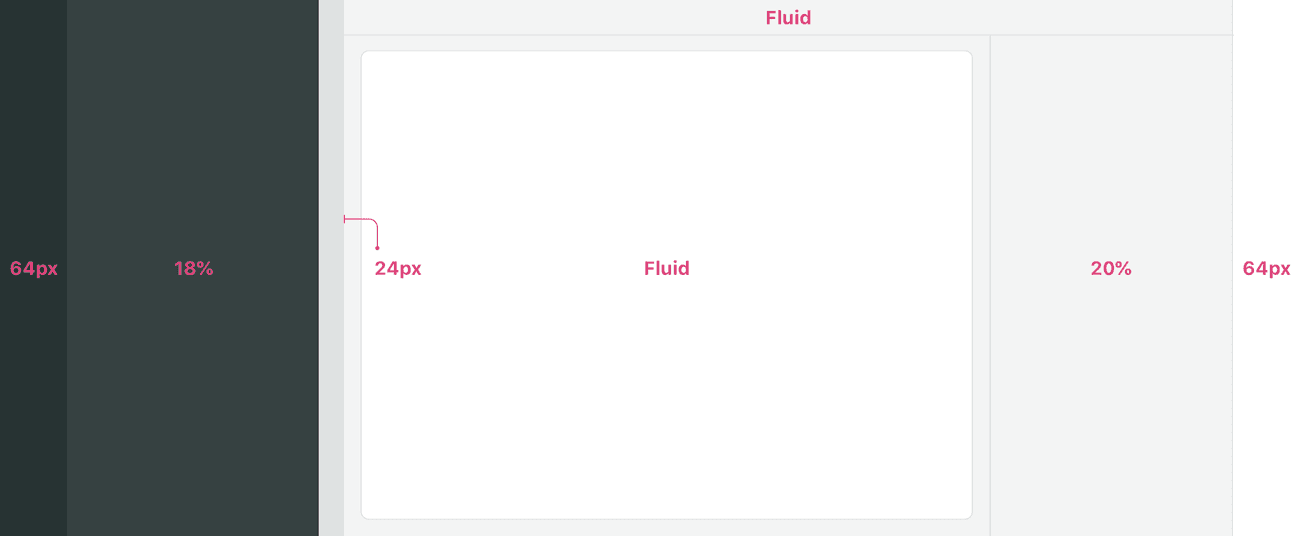This image showcases a composition of various squares and rectangles aligned side by side, each detailed with specific measurements and annotations:

- On the far left, there's a tall, vertical black rectangle. In the center of this black rectangle, "64 PX" and "18%" are displayed in red text.
  
- Right next to this black rectangle is a large white square. Midway along the left side of this square, "24 PX" is written in red text. Additionally, the word "Fluid" is prominently displayed with a capital "F" in red text to the right of the "24 PX" annotation. A thin, red arrow extends from the outer left side of the white square and points inward to the "24 PX" marking.

- On the far right of the composition stands a tall, vertical gray rectangle. Central to this gray rectangle, "20%" is inscribed in red text. Outside the rectangle, in the right-hand margin area, "64 PX" is marked in red text, indicating additional spatial information.

- Encompassing the large white square is a bigger, pale gray rectangle. At the top of this pale gray rectangle, the word "Fluid" is written in red text with a capital "F."

The red annotations and arrows emphasize important measurements and labels, providing clarity and context to the spatial relationships and dimensions of the elements within the image.